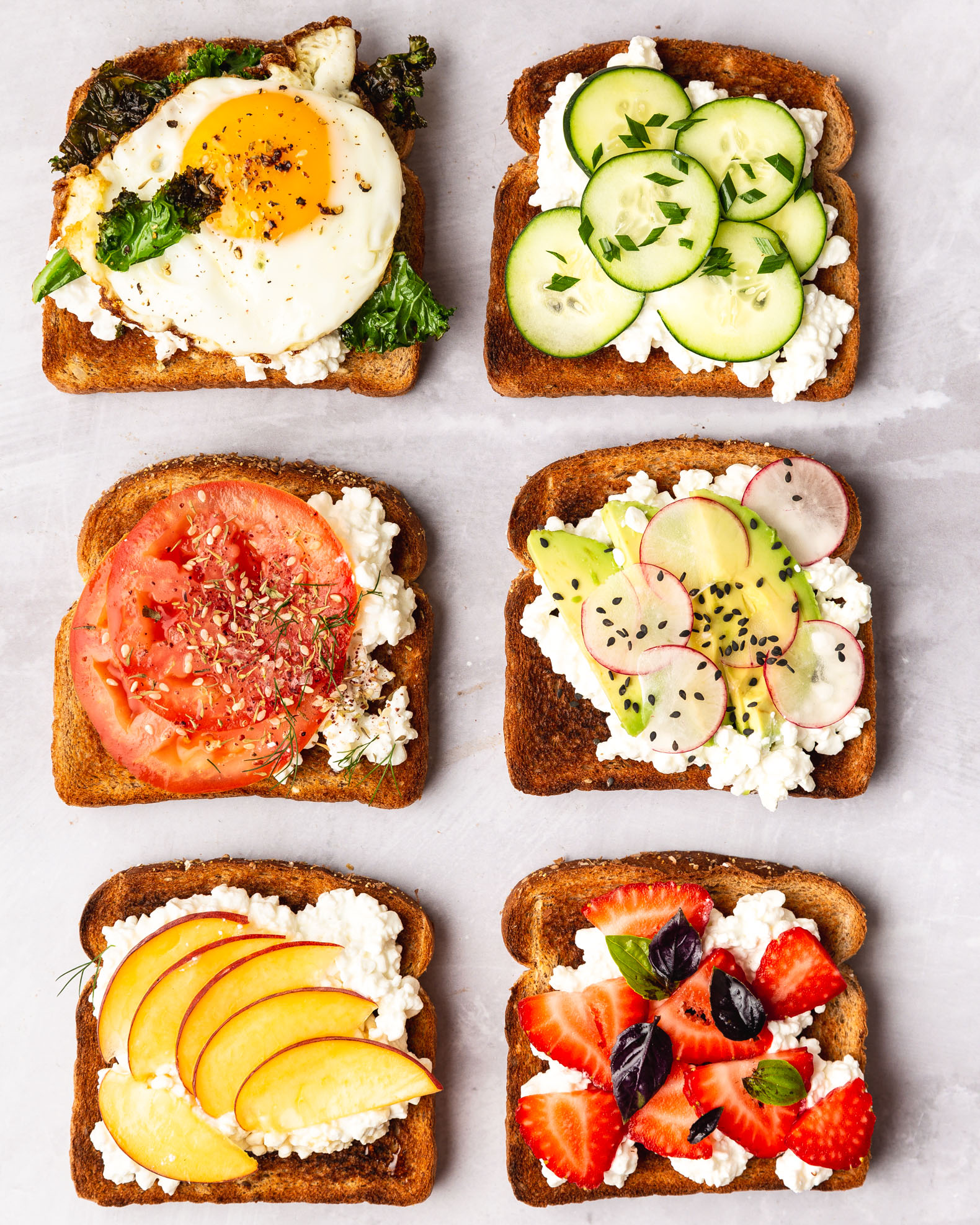The image showcases six pieces of toast arranged in a visually appealing grid pattern on a white marbled countertop. Each piece of toast features a unique and delicious topping. Starting from the top left, the first toast is adorned with an over-easy egg and a bed of dark green spinach. To the right, the second toast boasts slices of cucumber atop creamy cottage cheese. In the middle row, the left toast presents vibrant tomato slices seasoned and laid on cottage cheese, while the right one displays radish slices garnished with black seeds, possibly poppy seeds, on a spread of cottage cheese. The bottom left toast features peach slices arranged over a layer of cottage cheese, and the bottom right toast is topped with beautifully sliced strawberries and dark leafy greens. The toasts are all made from brown, sliced bread and are meticulously placed in two vertical rows of three, creating an enticing array of open-faced sandwiches that highlight a variety of flavors and textures.